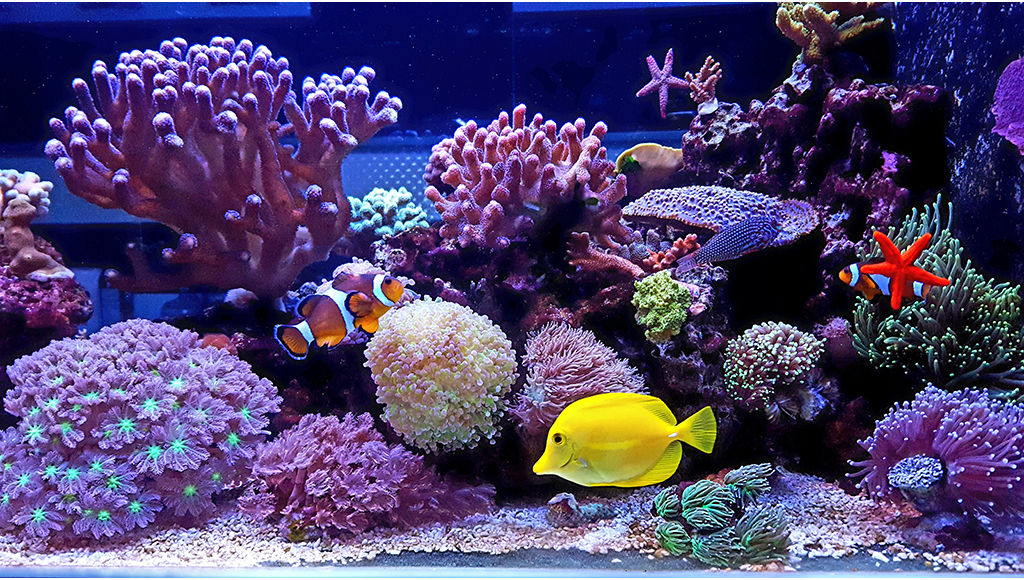This image showcases a vibrant saltwater aquarium, potentially located in a home or a public aquarium. The scene is bustling with diverse marine life and colorful underwater foliage illuminated by an ambient blue light. Prominently featured is a bright yellow tang swimming near the bottom right of the tank, difficult to miss with its vivid hue. Nearby are two distinctive orange and white clownfish, exploring their surroundings among anemones. 

The aquarium also hosts several starfish: a striking neon orange-red one seemingly attached to the side of the tank, and a purple starfish positioned towards the back. The bottom of the tank is decorated with white gravel and adorned with a variety of corals, ranging in colors from bright purples to greens, some of which may be fossilized. A mix of long, purple and pink sea plants adds to the lush underwater display, enhancing the tank's ecological diversity. The intricate plant and coral life not only provide a captivating visual appeal but also create a thriving habitat for the assorted marine species.